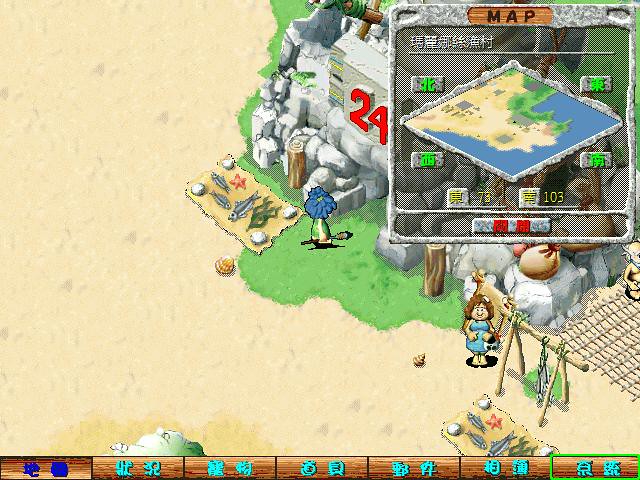This image is a screenshot from a low-resolution, browser-based video game, reminiscent of classic online games. The setting features a sandy area occupying the top right corner of the screen. Adjacent to this sandy terrain is a grassy section housing a stone structure with an archway, marked by the number "24" in red above it. In front of this stone structure lies a mat displaying an assortment of fish and other sea creatures. An identical mat with similar sea creatures is placed at the bottom right corner of the image, accompanied by some netting and a small wooden stand. 

Near the stand, a small female character is depicted, characterized by her brown hair and blue dress. A sizable map is displayed at the top right corner of the screen, revealing the surrounding area where the character is located. All the in-game text, except for the word "map," is in Chinese, including the buttons arrayed along the bottom of the screen. This screenshot captures a moment rich in detail, reflective of casual exploration or a marketplace setting within the game.